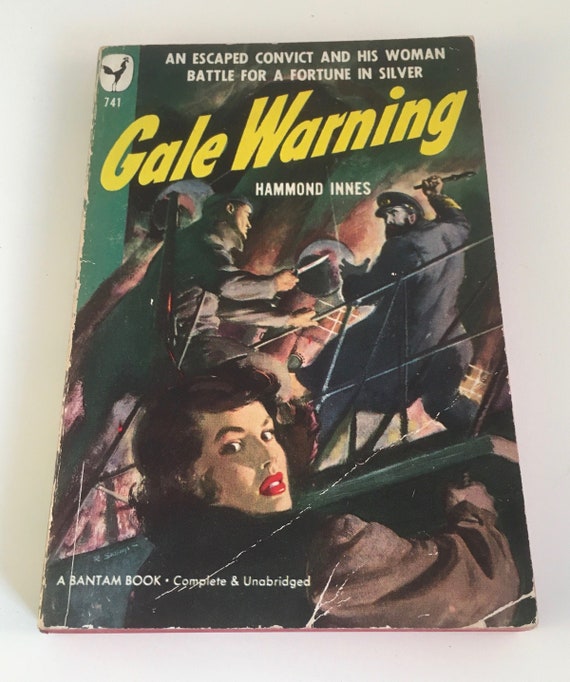The image showcases a vintage paperback book with a distinct film noir aesthetic, evident from the creases in its cover. At the top of the book, in white print, the tagline reads, "An Escaped Convict and His Woman Battle for a Fortune in Silver." Below this, the title "Gale Warning" is prominently displayed in bright yellow letters. The author, Hammond Innes, is credited just beneath the title. The illustration on the cover depicts a dramatic scene: a woman, who appears worried, is grabbing onto something while looking back over her shoulder. She has dark, wavy shoulder-length hair, bright red lipstick, and is dressed in a brown coat. Two men are engaged in a fierce struggle; one, clad in coveralls with a knife in hand and a shotgun slung across his back, and the other, in a gray suit wielding a pipe wrench. Printed at the very bottom in white is a note that this is "A Bantam Book, Complete and Unabridged."